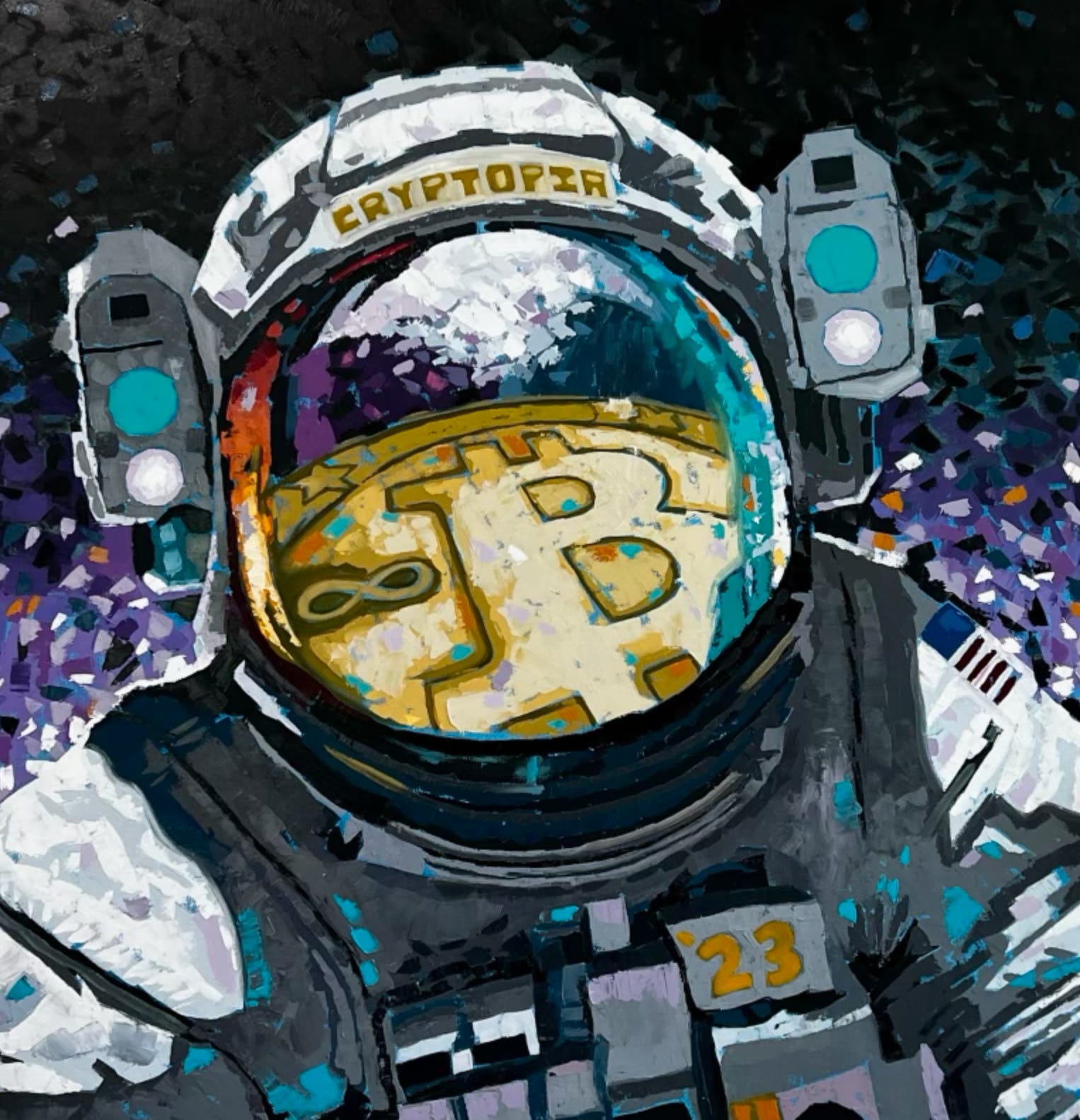The image is a highly detailed painting of an astronaut in a white and gray spacesuit, surrounded by a vibrantly colored space scene. The astronaut's visor is down, reflecting a large, gold Bitcoin coin adorned with stars on its rim and an infinity symbol to the left, alongside the distinctive Bitcoin logo with a 'B' crossed by two vertical lines. Above the visor, the word "CRYPTOPIA" is inscribed in gold lettering. The suit features the number "23" in gold on the left chest area. The helmet is equipped with two mounted lights or cameras on either side. The background transitions from black at the top to a mix of white, black, purple, magenta, light purple, and orange hues in the middle, creating a dramatic celestial atmosphere. The intricate detail and rich colors weave together to craft a mesmerizing and vivid depiction of an astronaut in space, exploring the digital realm symbolized by the Bitcoin reflection.